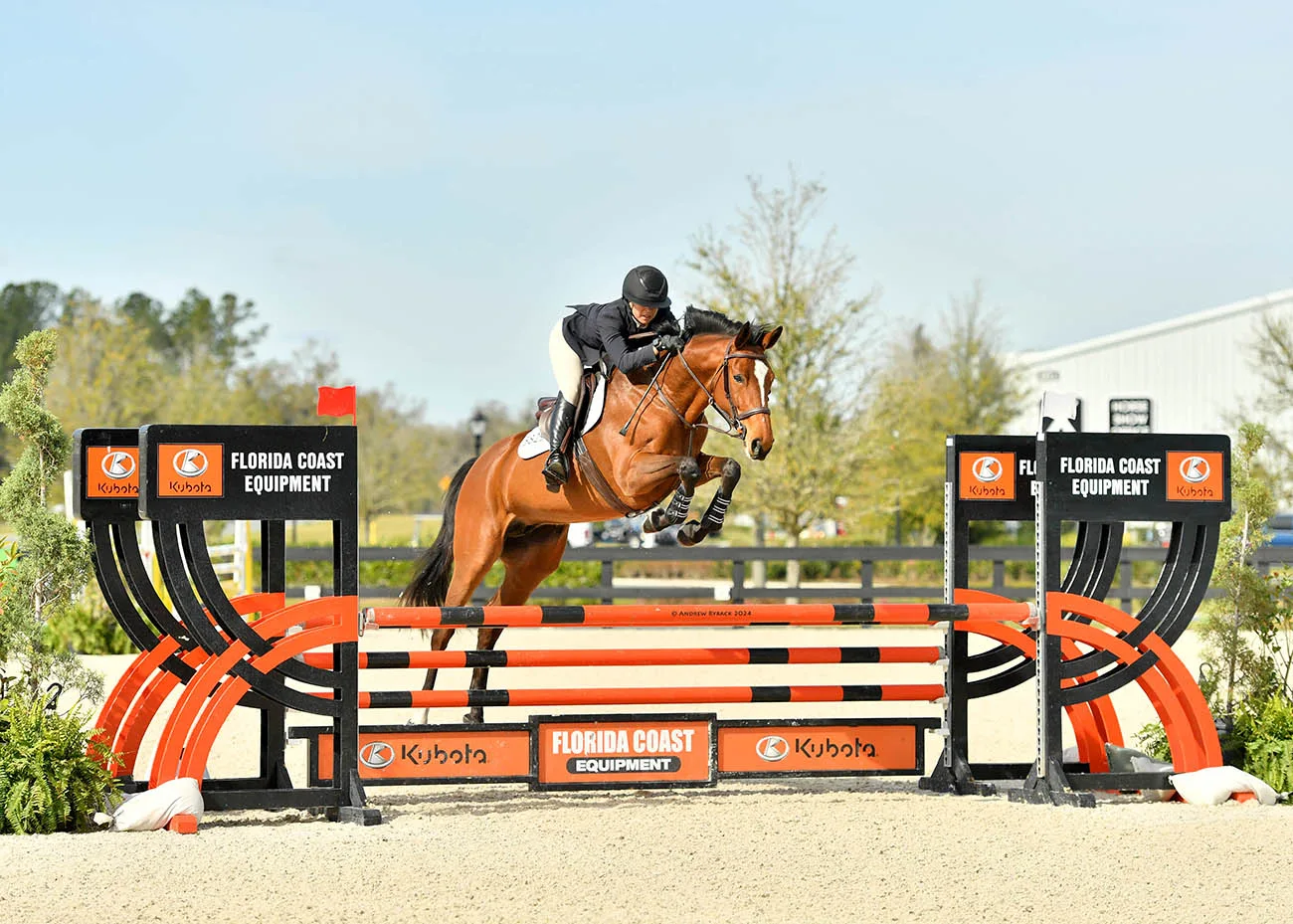This detailed action photograph captures a jockey riding a stunning, caramel-colored brown horse with a shiny coat, black mane, and tail. The horse is in mid-air, slightly less than halfway over an obstacle with three horizontal bars, which are orange with black stripes. The jump prominently displays the text "Florida Coast Equipment." The jockey, dressed in a black long-sleeved jersey, black helmet, black boots, and white pants, is perfectly positioned atop the leather saddle. The setting is a dirt course composed of sand or small rocks, surrounded by green trees and a white building to the right. Above, the sky is a clear, vibrant blue, contributing to the natural brightness and clarity of the image.